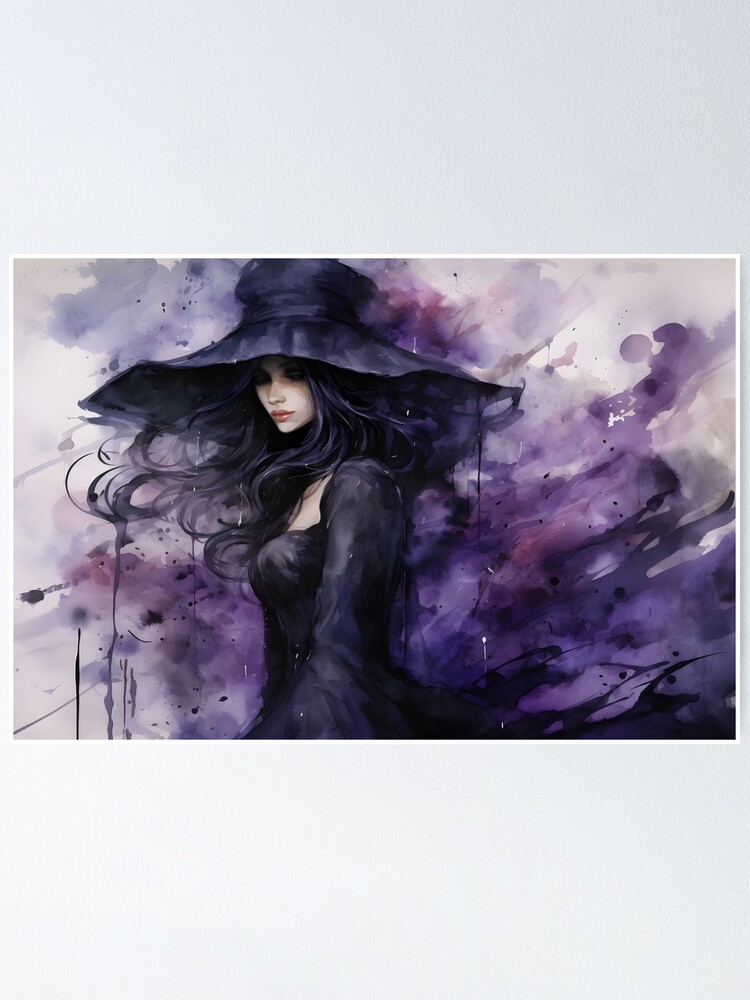The image depicts a painting of a young woman centered slightly to the left. She has a very angular, pale white face accentuated with large lips painted in lipstick and darkened eyes, which are partly shadowed by an immense, black hat with a poofy round top and a belt around it, wide enough to resemble an umbrella. Her hair is a wild, wavy mix of blue or bluish-black, cascading chaotically around her. She is dressed in a long-sleeve black dress, low-cut over her chest, which gets cropped at her waist. The entire scene is enveloped in a dynamic swirl of watercolors, predominantly purples and blacks, giving a sense of fluidity and motion. Light purples, white, and beige accents, along with streaks resembling water stains, add texture and depth to the background. The painting is framed by a white border and set against a grey background, creating a striking contrast that highlights the vividness of the watercolor elements. The style suggests a modern interpretation of a witch, rich with subtle yet intriguing details.